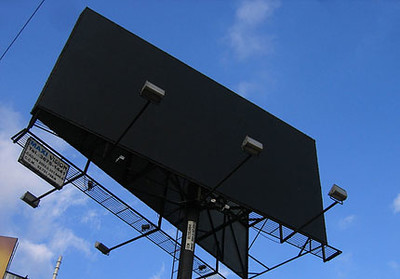Under a vivid blue sky dotted with wisps of white clouds on the left, a prominent billboard stands at the center of the scene. The billboard is mounted on a tall pole and features three protruding lights, suggesting it is designed to be illuminated at night. Below, there is a platform, likely used for maintenance or changing the billboard's display. The current ad on the billboard bears the text "MaxiVision" amidst other textual content. To the bottom left, the edges of another billboard are visible, characterized by a distinct yellow border. This second billboard also appears to have lights aimed at it, probably to enhance visibility.